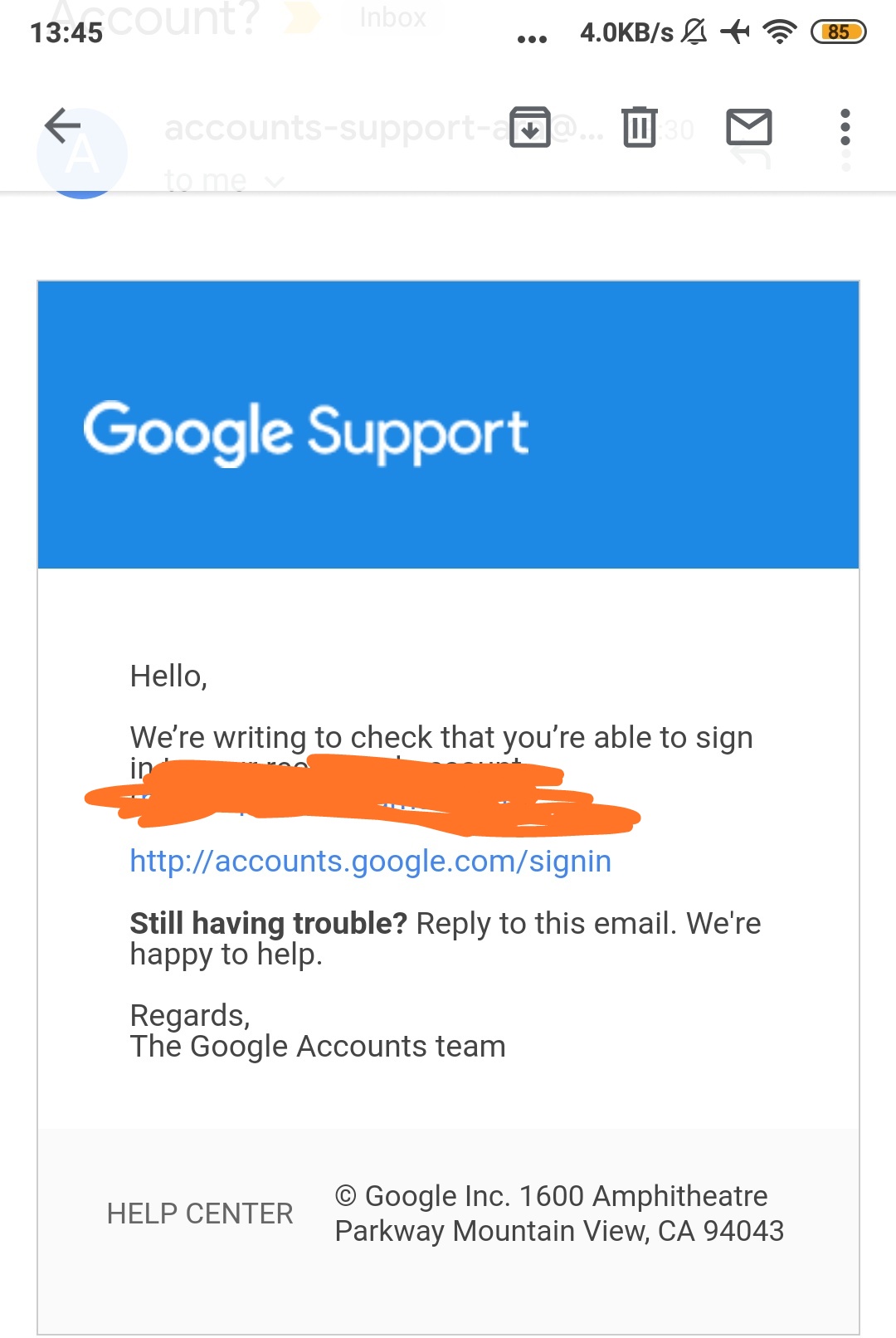The image depicts a cell phone screen showcasing an email from Google Support. The screen's top left corner displays the time, 13:45, along with three horizontal dots, a data usage of "4.0 KB/s", a notification bell icon indicating notifications are off, an airplane mode icon, a battery indicator at 85%, and a Wi-Fi signal icon. Below these indicators, there is a toolbar with four icons: a left arrow, a mail icon, a trash bin, and a "move to file" icon.

The email header is set against a blue background with the text "Google Support" in white. Beneath this, the email body starts with the text on a white background: 

"Hello, we're writing a check that you are able to sign," followed by a section of the sentence that is scribbled out in orange. The email includes a call to action directing the recipient to "http://accounts.google.com/signin" and offers further assistance by replying to the email with "We're happy to help. Regards, the Google Accounts Team."

At the bottom of the email, it shows a footer with "Help Center" and the company details: "© Google Inc., 1600 Amphitheatre Parkway, Mountain View, CA 94043." The email interface and content display a combination of orange, blue, black, gray, white, and yellow colors.